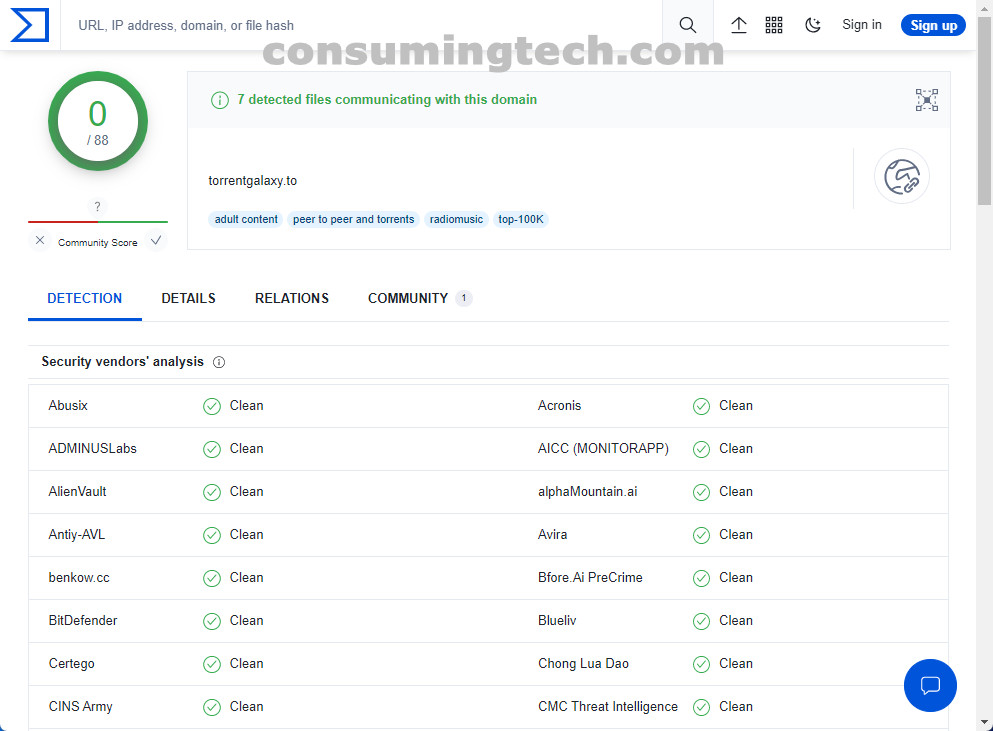The image displays a webpage with various details. At the top of the page, there is a blue banner resembling a flag with stripes, situated horizontally like a crown. The banner includes the words "URL," "IP address," and additional text, all in gray. Centrally positioned is the site name, "consumingtech.com," appearing in gray font. Above this name, there are options to sign in, sign up, and several other navigation links.

Beneath this section, dominating the page is a large green circle. Within this circle is a large white zero, followed by the number 88 directly underneath it. The text below the circle indicates "7 detected files communicating with this domain," alongside classifications such as "Foreign," "Torrent Galaxy 2," "adult content," "peers," "peer-to-peer and torrents," "radio," "music," and "top 100,000."

To the right of this section, there is a monochrome image of the globe. The webpage content is organized into columns labeled "Detection," "Details," "Relations," and "Community," with the "Detection" tab currently highlighted. The "Community" tab displays a number 1, indicating a single notification or message.